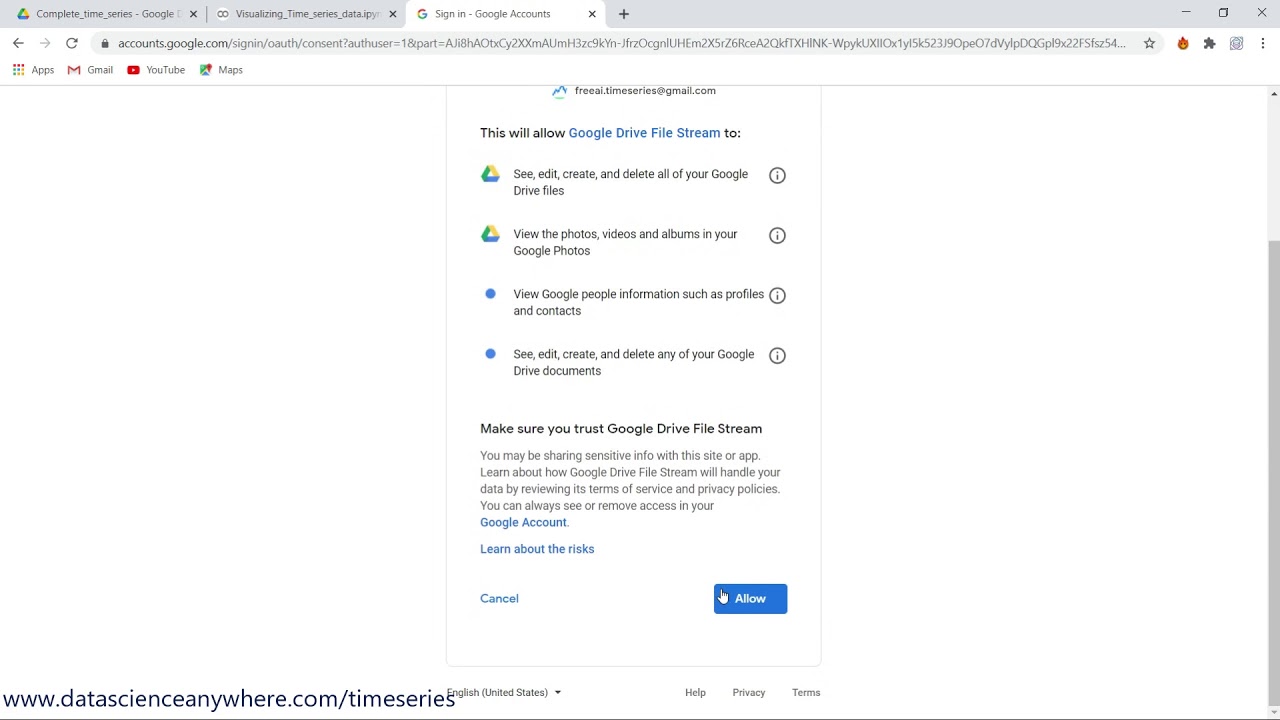The image is a screenshot of a Google account authentication page set against a mostly white background. At the top of the page, there's a gray border featuring multiple tabs, with the active tab labeled "Sign in - Google Accounts." Below this border, the address bar is visible, displaying a URL beginning with "accounts.google.com" followed by a lengthy string of characters and numbers that stretches across the page.

Directly beneath the address bar are various icons, each representing different Google services including Apps, Gmail, YouTube, and Maps. The focal point of the image is a central box containing detailed permission information. The text within this box indicates that Google Drive File Stream will be granted the ability to see, edit, create, and delete all Google Drive files, view Google Photos (including photos, videos, and albums), and access Google People information such as profiles and contacts. Additionally, it outlines permissions to see, edit, create, and delete any Google Drive documents. Each permission item is accompanied by an icon depicting an eye inside a circle.

The text also advises the user to ensure they trust Google Drive File Stream, as sensitive information may be shared with this site or app. It suggests reviewing the terms of service and privacy policies to understand how Google Drive File Stream will handle the user’s data. An advisory note mentions that users can always manage or revoke access within their Google account. Below this text, there are options to "Learn about the risks," "Cancel," and "Allow," with the cursor—a person's hand—hovering over the "Allow" button.